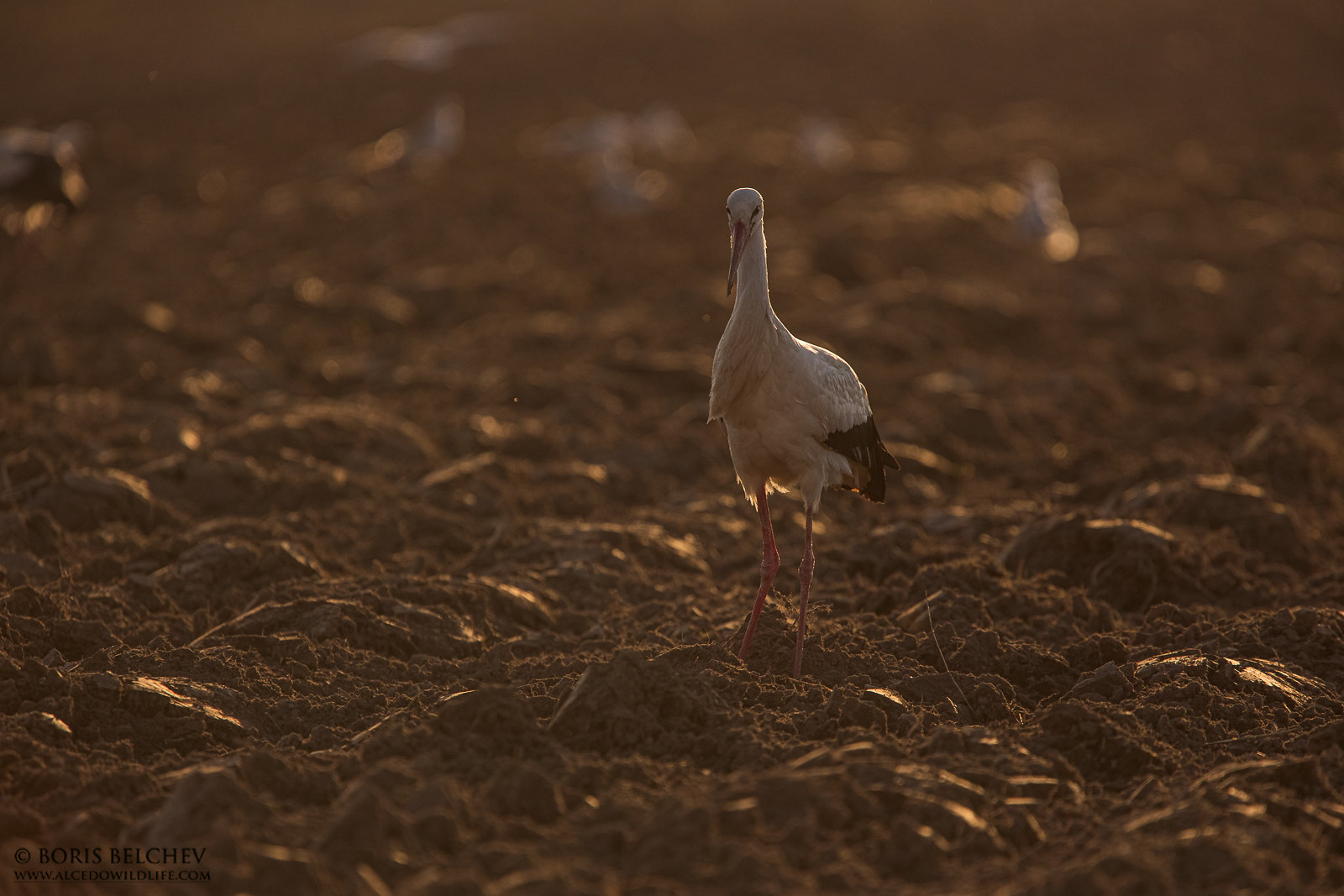In this dusk-lit photograph, the focus is drawn to a solitary crane standing in freshly tilled, loose brown soil, interspersed with various strands of vegetation and roots. The bird has long, skinny orange legs that blend into the dirt, obscuring its feet. The bird's body is primarily white, with some gray feathers mixed in, and contrasted by its black wing edges and black tail feathers. The crane's most striking features are its long, pointed orange beak and its two small black eyes, which gaze forward. In the lower portion of the image, the name "Boris Belchev" along with the website "www.alcedowildlife.com" is visible. The background, though dark and somewhat out of focus, shows a continuous expanse of the same freshly turned brown soil, providing a consistent and natural setting for the bird.